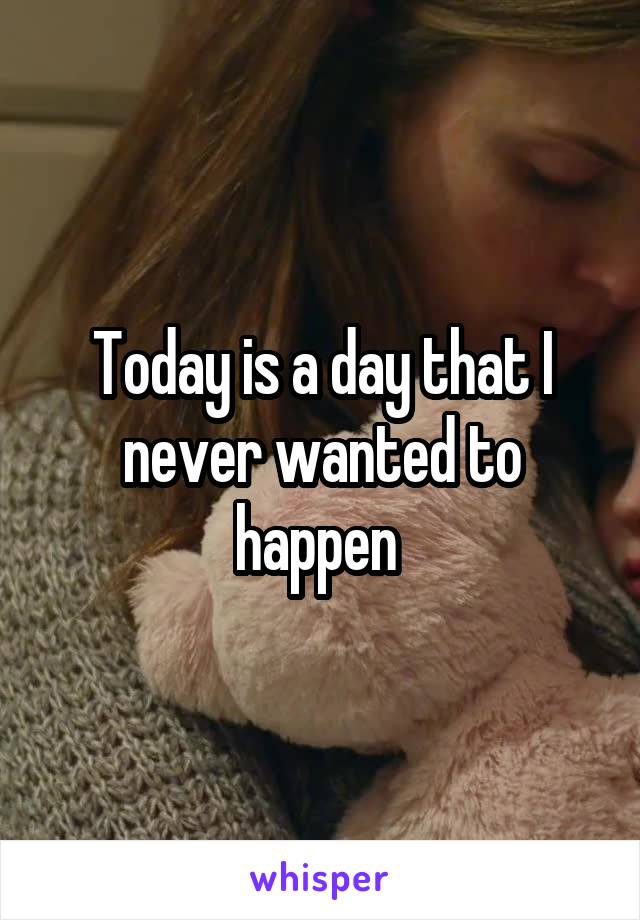The image is a meme-style photo featuring a sad-looking white woman with long brown hair, wearing a gray sweater. She is holding a young child on her left arm and a pink teddy bear in her right arm, with only the backside of the teddy bear visible. The woman is looking downward, appearing somber, with the child partially cut off on the right side of the image. The background includes a textured element, possibly a headboard. Across the center of the image, there is white text that reads, "Today is a day that I never wanted to happen." At the bottom, in lowercase purple letters, the word "whisper" is displayed. The overall aesthetic suggests a poignant or motivational message intended for social media sharing.